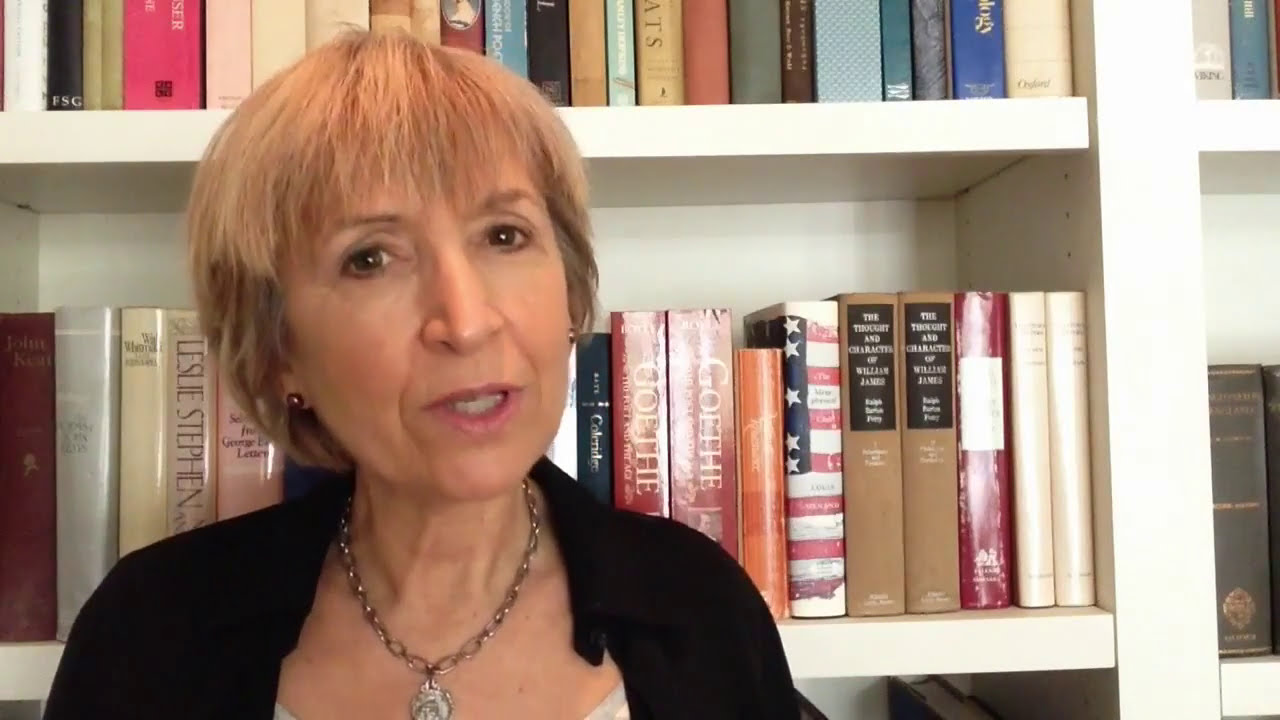In the image, an elderly woman sits slightly off-center to the left, gazing intently into the camera with her lips parted as though she's speaking, suggesting an interview setting. Her short hair is a mix of light brown and blondish gray, and her dark brown eyes stand out against her fair skin. She wears a black sweater over a lighter-colored blouse, accompanied by a notable silver chain necklace with an ornate, round pendant. Her attire is simple yet expressive, with small stud earrings visible on her ears.

The backdrop features a white bookshelf filled with neatly arranged hardcover books of various colors, including white, black, green, pink, brown, light blue, dark blue, red, and silver. Specific titles and notable book covers are discernible, such as a collection of stories from William James and books by Leslie Stephen. There's also a book designed to resemble the American flag with red and white stripes and a blue section adorned with white stars. The light-colored shelves themselves add to the impression of a well-kept, organized space, possibly within a library or a personal home library. The woman's intense expression combined with the scholarly setting gives the image a poignant, thoughtful quality.